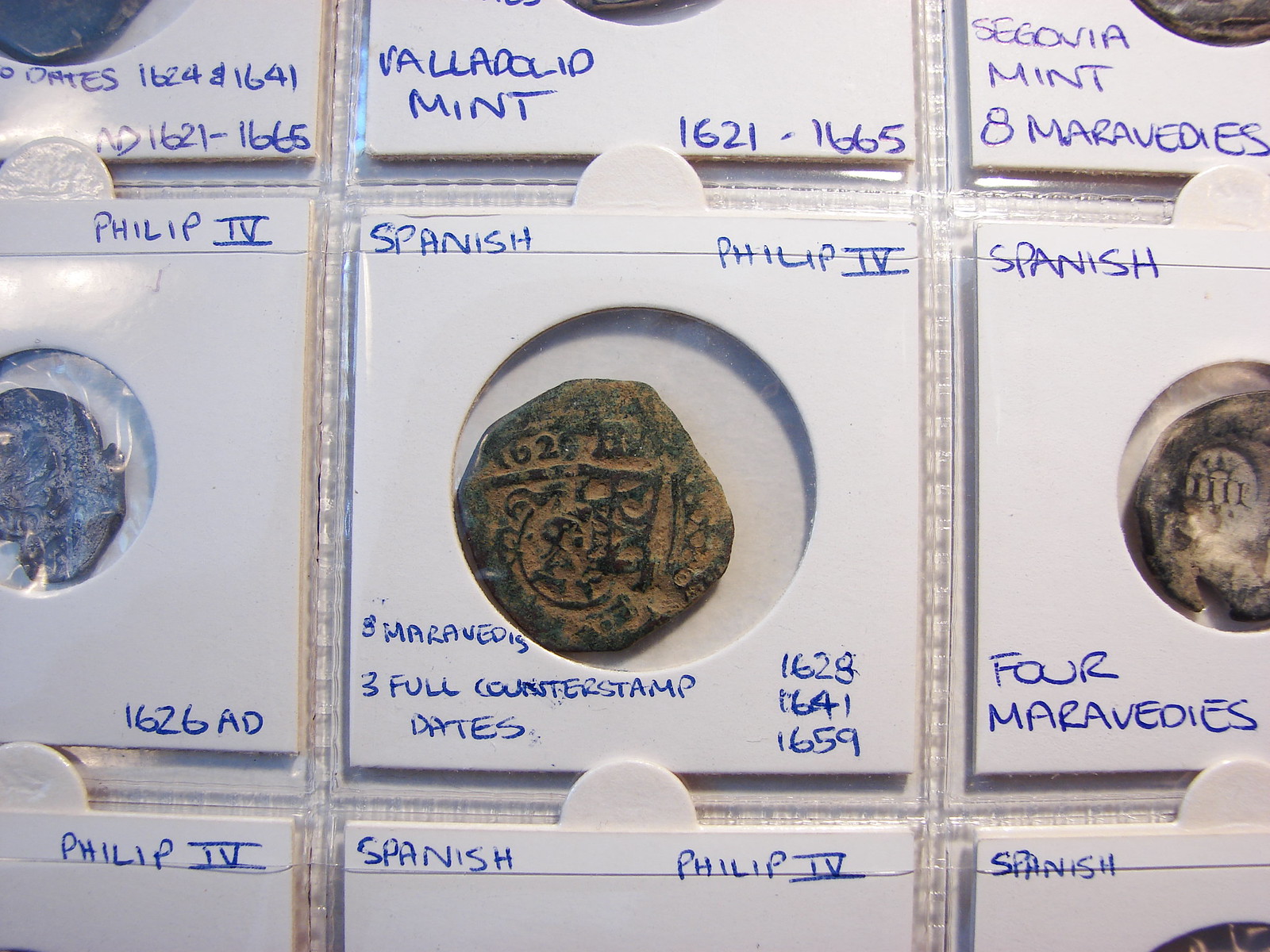This detailed image showcases an antique coin collection meticulously preserved and categorized within a 3x3 grid display book. Each of the nine slots contains a unique coin, with particular emphasis on their historical value and origin. The centerpiece is an especially notable Spanish coin from the era of Philip IV, displaying three distinct counter stamp dates: 1628, 1641, and 1659. This coin, housed in a white sleeve, exhibits a brownish dark gray hue with a worn texture and a greenish substance. Handwritten blue inscriptions on the sleeve detail "Spanish" in the top left corner, "Philip IV" on the top right, and "Three Maravillas" alongside the counter stamp dates. 

Surrounding this centerpiece, other coins share similar antique characteristics, often with irregular shapes and worn surfaces. Notable mentions include:
- The slot above the center, labeled "Valladolid Mint" and dated 1621 to 1665.
- The slot to the right of the center, labeled "Spanish" and "Four Maravillas," showcasing another worn and uniquely shaped coin.
- Various other slots containing partial inscriptions and dates, such as "Segovia Mint" and a mix of dates ranging from 1621 to 1665.

Overall, the collection reflects a significant historical period through its carefully labeled and preserved coinage, providing a fascinating glimpse into the past.